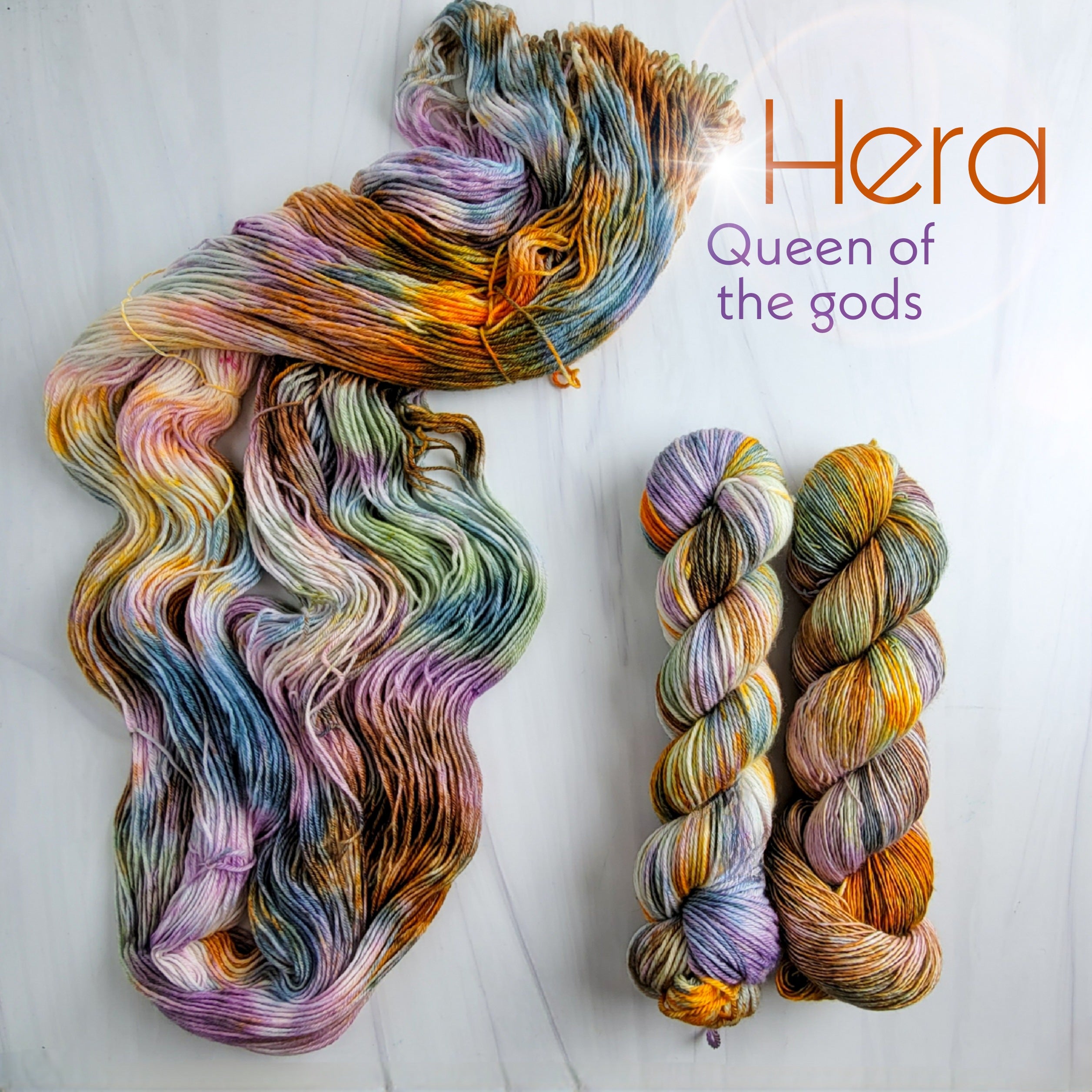The image depicts three multicolored ropes, intricately woven from numerous strands, creating a thick and textured appearance. The vibrant ropes exhibit a spectrum of colors, including faded purples, blues, greens, and oranges, evoking a rainbow-like effect. Two of the ropes are neatly knotted, while the third remains partially unraveled, enhancing the visual interest of the composition. In the top right corner, a title reads "Hera, Queen of the Gods," referencing the Greek goddess Hera.